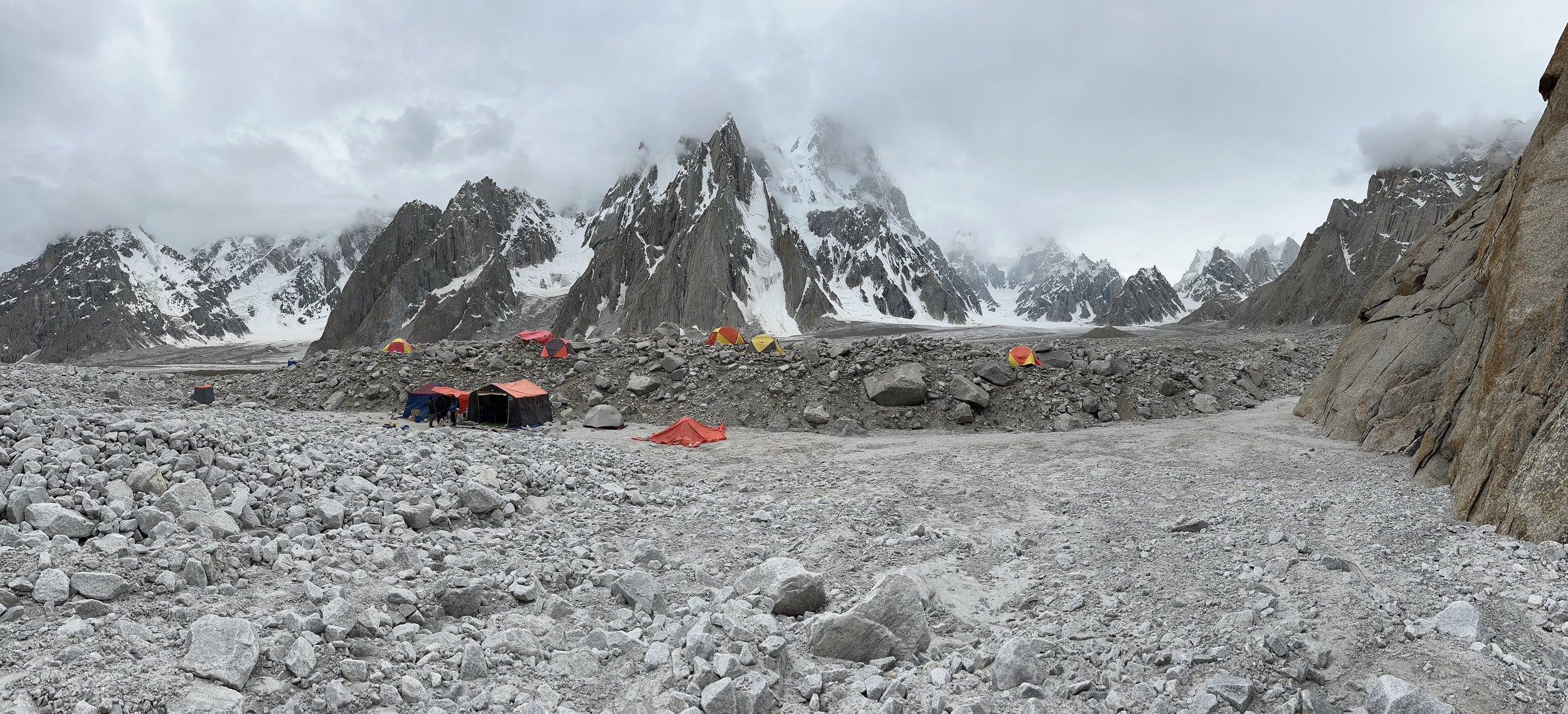The image captures a rugged mountain landscape, featuring a campsite amidst a desolate, rocky terrain. The ground is predominantly gray, scattered with numerous rocks and patches of dirt, devoid of any vegetation. In the background, there are towering mountain peaks that exhibit a dark brown and gray hue, capped with patches of snow. The sky overhead is overcast, with clusters of fluffy clouds drifting near the mountain summits, adding a dramatic touch to the scene.

The campsite is comprised of several tents, each dispersed across the rough ground. Among them, a few tents stand out with red tops and black sides, while additional tents display vibrant shades of yellow and orange. Two of the tents, positioned side by side, appear larger than the others, suggesting they might be the central hub of the camp. There are a few figures visible in front of these larger tents, possibly engaged in setting up or interacting at the campsite. The overall atmosphere is stark and remote, emphasizing the raw beauty and challenging conditions of this high-altitude wilderness.